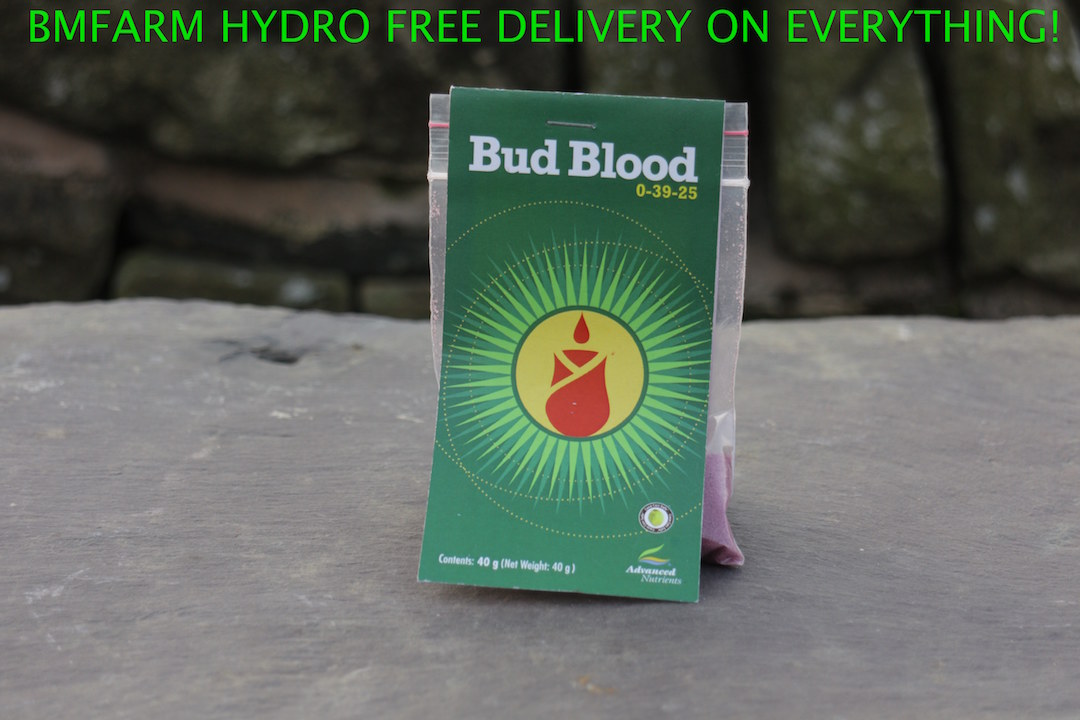The photograph captures a green package labeled "Bud Blood 0-39-25," resting on a grey stone surface. The package is a plastic Ziploc bag with a printed label stapled around it, obscuring its contents. The prominent label features a yellow circle with a red candle illustration surrounded by green rays, evoking a star shape. In the lower right corner, the label reads "Advanced Nutrients," while the bottom left corner states the weight as "40 grams." Additionally, the top of the label displays the text "BM Farm Hydro Free Delivery on Everything!" The background consists of a wall made of stacked stones, providing a rustic texture to the setting.